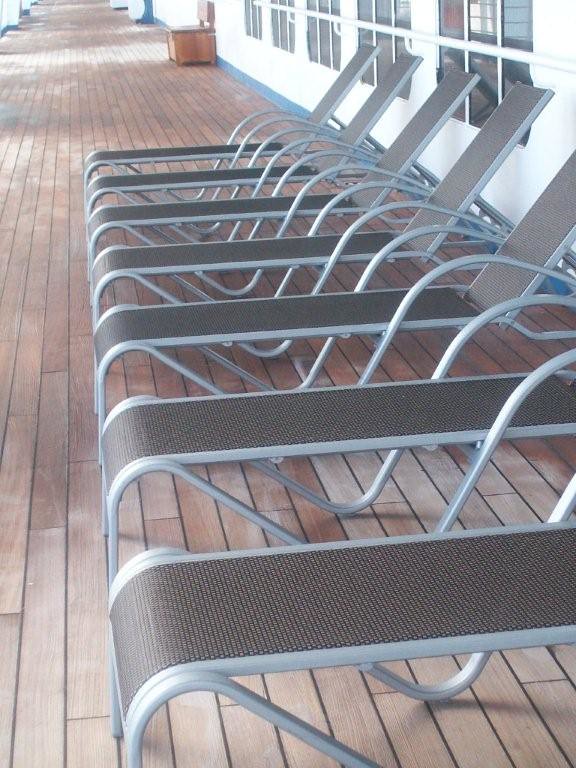The image depicts what appears to be the deck of a cruise ship, characterized by its brown wooden flooring. Along the right-hand side, there are seven identical chaise lounge chairs made of silver metal with woven brown seating that extends into a long backrest. These chairs line up against a white building with blue trim, which features a series of five sets of windows. The building, resembling typical cruise ship architecture, also has a railing running along it. A wooden box—potentially serving as both a seat and storage—sits slightly further up from the chaise lounges. The overall perspective of the photo suggests that this deck extends for quite a distance, although it is cut off in the image. In the upper left corner, there appears to be a walkway and hints of a body of water, enhancing the outdoor maritime ambiance of the scene.